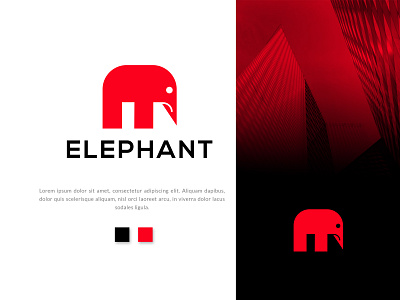This image appears to be an advertisement or business card, characterized by a striking, split design. The left side features a white background with a prominent red elephant logo, which is a simplified, symbolic drawing showing only essential elements like eyes, a pointy trunk, and legs. Above the logo is the word "ELEPHANT" in bold, black, uppercase lettering, and below it is an unreadable blurb of text. Two small adjacent boxes—a black one and a red one—are positioned beneath the text. The right side is starkly different, presenting a gradient background that transitions from deep black at the bottom to vivid red at the top. This side showcases another red elephant logo, somewhat smaller, set against a complex geometric pattern including an upside-down V shape and a red lattice-like design. Together, the composition employs a limited but impactful color palette of white, red, and black, enhancing the visual appeal and symmetry of the overall design.